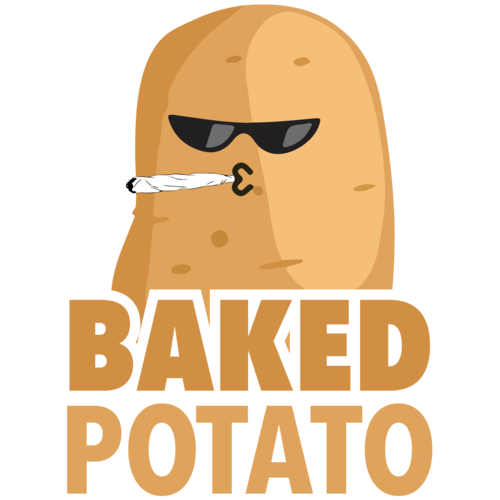The image features a cartoonish potato rendered in three different shades of brown, giving it a textured appearance. The potato is anthropomorphized with black aviator-style sunglasses perched on its face, though no sides to the glasses are visible. Below the sunglasses, the potato has a slightly curved, black mouth, which is clasping an unlit joint. The background of the image is plain white. At the bottom of the image, occupying almost half of the total space, is the text “baked potato” written in varying light and dark brown shades. The overall humor of the image suggests a play on words, implying the potato is "baked" or high, making it resemble a meme.